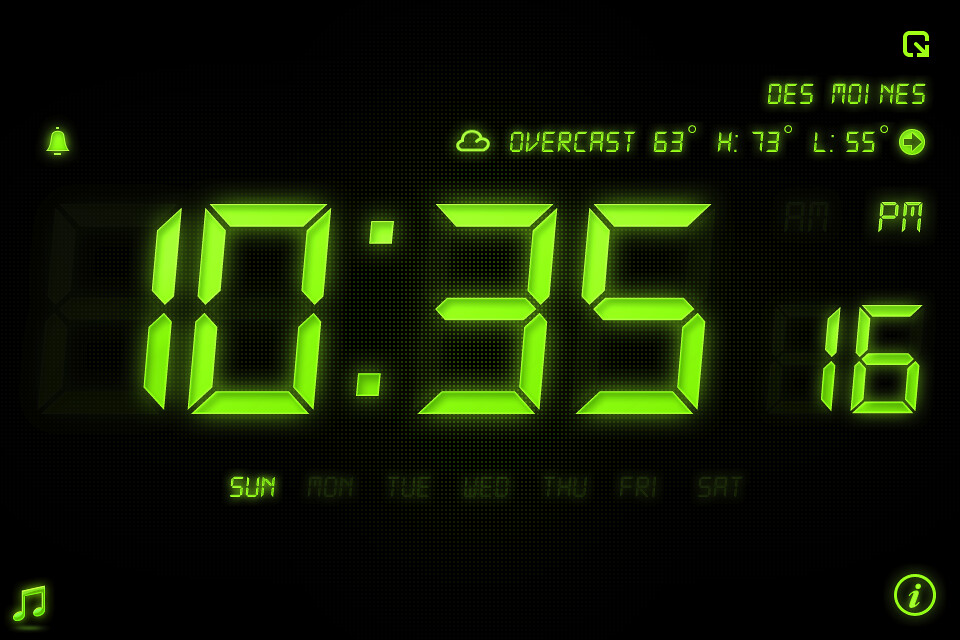The image is a screenshot of an alarm clock app's LCD screen on a phone. The display has a crisp, clear quality with a plain black background. The time shown is 10:35 PM and 16 seconds, with the day of the week, Sunday, highlighted at the bottom among all days of the week. The text on the screen is neon green. In the top left corner, there is a small alarm bell icon, while in the top right corner, an exit or minimize button is visible. The screen also shows weather information, with a cloud symbol indicating overcast conditions directly above the "35" in the time. The temperature reads 63°F, with a high of 73°F and a low of 55°F. The information includes the location, DES MOINES, displayed in yellow text. In the bottom left corner, there is a music note icon, and in the bottom right corner, an information icon.